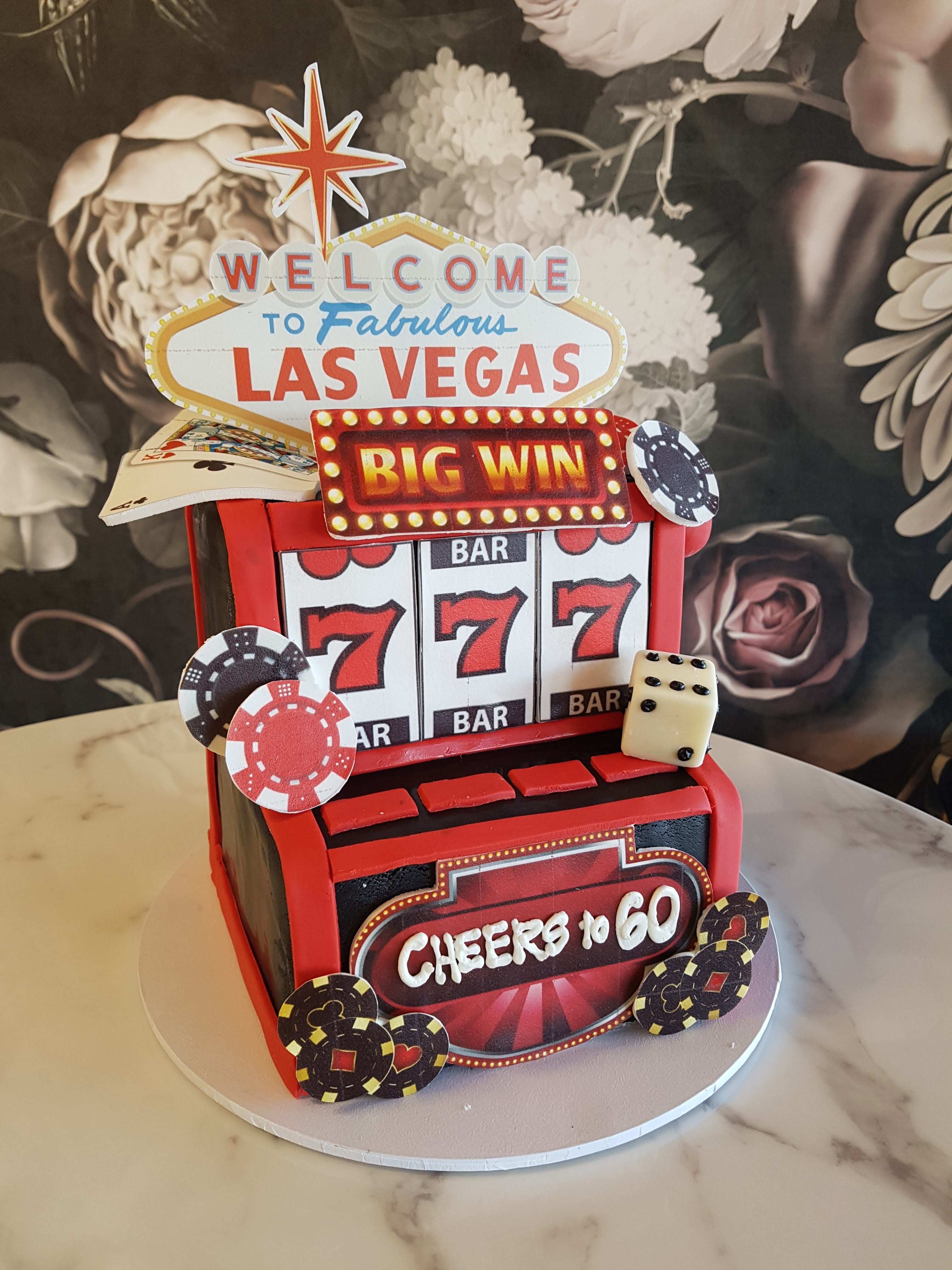The image showcases an intricately designed cake that resembles a slot machine, placed on a white plate set on a round marble tabletop. The slot machine cake, with black sides trimmed in red, features the phrase "Cheers to 60" at the base in white letters. Above this, the context of a slot machine is detailed with four small red rectangular buttons and a screen with three red sevens (777) displayed prominently, indicating a win. At the top of the cake, the words "Big Win" are highlighted within a rectangle outlined in light bulbs. To the right of this, a poker chip is visible. The left side of the cake features a stack of poker chips, while the right side showcases a single die. Additionally, the left part of the cake is adorned with two poker chips. Above the central screen, there are cards featuring an ace of clubs and a king of hearts bending to the left. Sitting atop the cake is the iconic “Welcome to Fabulous Las Vegas” sign complete with its signature red star. The background of the image includes a wallpaper with painted flowers in shades of gray, white, and light pink, enhancing the celebratory theme.